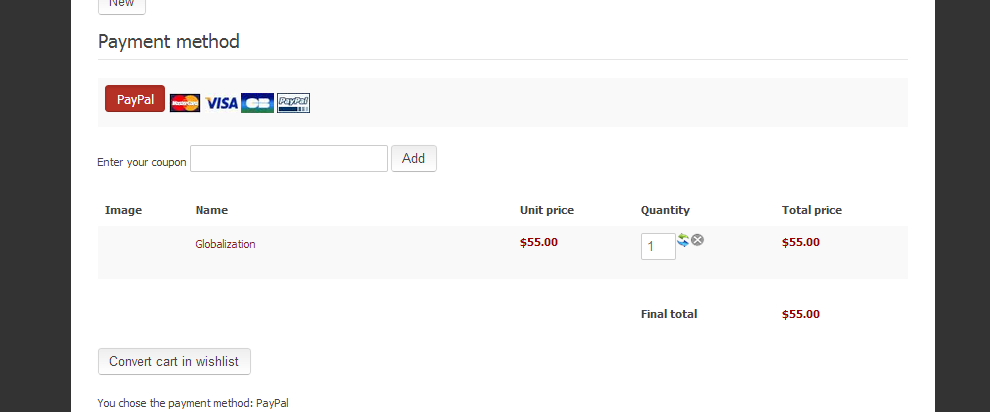This cropped screenshot depicts a payment page for a product from an unidentified storefront. At the top of the page, a partially visible button labeled "New" can be seen. Below it, the payment methods available are listed, including PayPal, MasterCard, Visa, an unclear option that might be "GB" or "CB," and another PayPal option, with PayPal currently selected.

There is a section dedicated to coupon entry, featuring an empty input field for coupon codes. Further down, the page displays columns for the product's name, unit price, quantity, and total price—though there is no accompanying image for the product. The product listed is named "Globalization" with a unit price of $55, a quantity of one, culminating in a total of $55. The final sum for the order is also $55.

Additional features on the page include buttons for converting the cart to a wishlist and options to choose different payment methods, with PayPal already chosen. The screenshot is noticeably cropped, with various elements partially cut off, and the page has a simple white background accented by gray bars separating different sections. There are also black bars on the left and right sides of the image. Given the product name, "Globalization," it may likely be a textbook or an academic course, although the exact nature is unclear due to the vague naming.